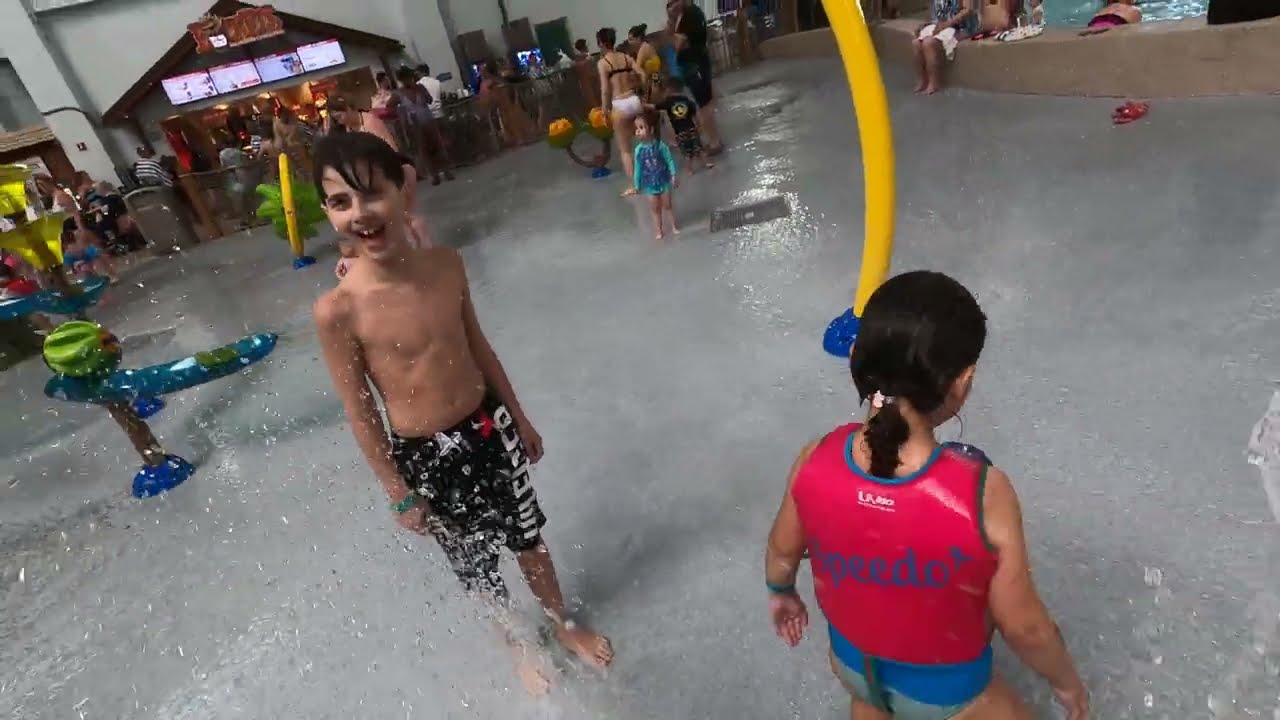The image depicts a vibrant indoor water play area within a mall, bustling with activity. Central to the scene is a young girl with brown hair, wearing a red Speedo life preserver jacket. Nearby, a boy in swimming trunks, also with brown hair, is enjoying the water features, smiling at the camera. The ground is wet and dotted with small fountains spraying water upwards, creating a whimsical atmosphere. Surrounding the children are various water play structures, including one with a spinable palm tree. In the background, multiple people stand or sit near a railing, observing the lively scene. Among the themed objects, tropical fruit designs such as melons, a banana with leaves, and a watermelon are embedded into the ground, enhancing the playful environment. A trash can is also visible outside near the railing area. The overall mood is joyful and dynamic, capturing the essence of a lively day at the water play area.